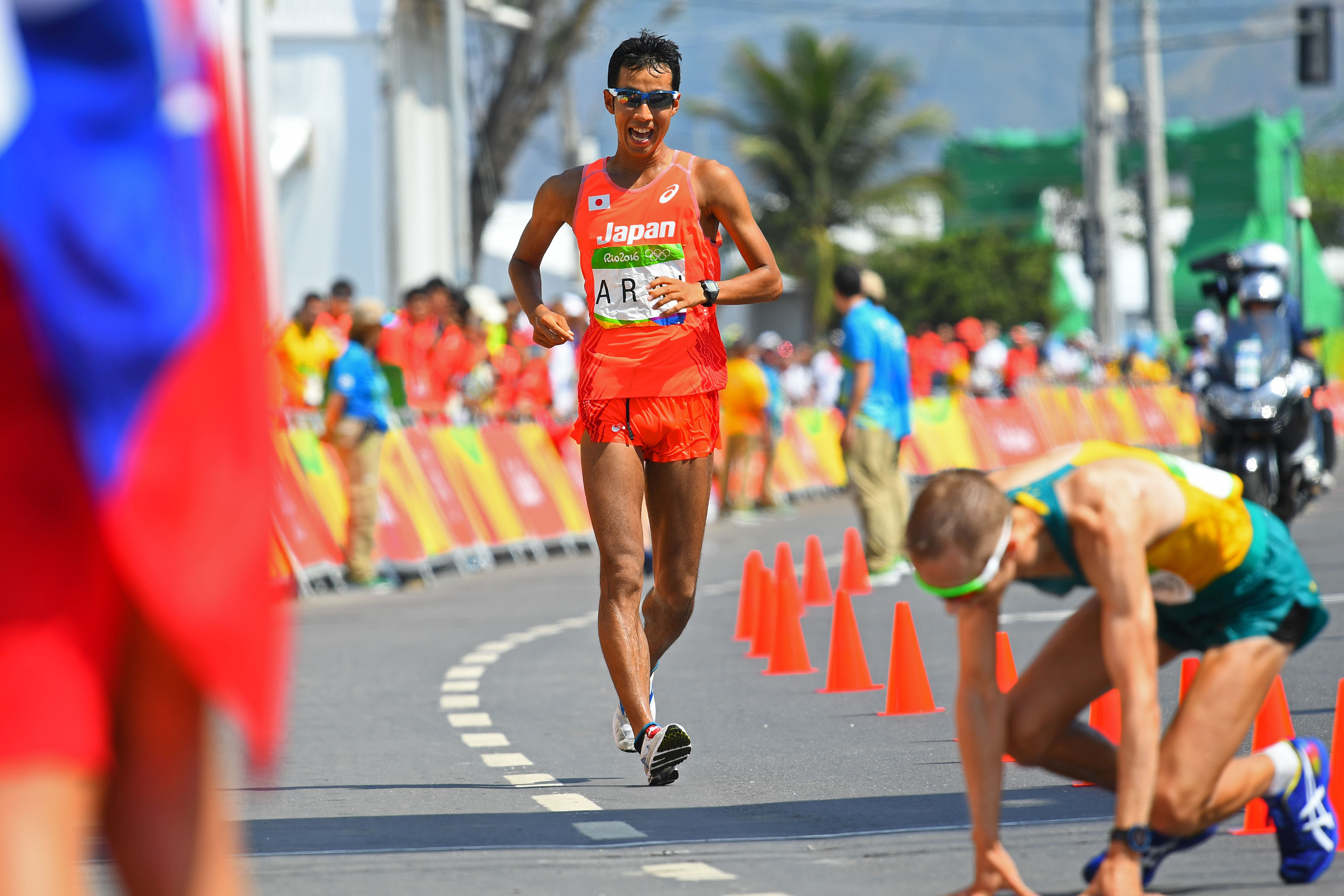This photorealistic image captures a vibrant and energetic race scene, focused primarily on an Asian man with dark hair, presumably Japanese, who is in mid-stride either running or walking. He is donned in an orange tank top and shorts, with the word "Japan" featured prominently in white across his chest, along with a racing number that is white and green. The setting is an outdoor race track, defined by its gray surface and marked with orange pylons on the right side to guide the runners. 

In the foreground, the Japanese man appears to be making significant progress, while another runner in a yellow and turquoise ensemble, wearing blue sunglasses, is seen kneeling or trying to rise from the ground nearby. This runner is described as balding and possibly having stumbled.

The background adds to the lively atmosphere, packed with spectators contained behind red and yellow stands. This colorful crowd indicates the support and excitement surrounding the event. To the right, a person on a silver motorbike, likely a cameraman, is capturing the race. Additionally, the scene includes some environmental details such as buildings, light posts, and greenery with a palm tree distinctly visible near the center. The left side of the image features another spectator, dressed in blue and red, though they are blurred due to the camera's focus on the foreground. The text "Rio 2016," hinting at an Olympic event, is visible on the athletic apparel, emphasizing the competitive, international nature of the race.